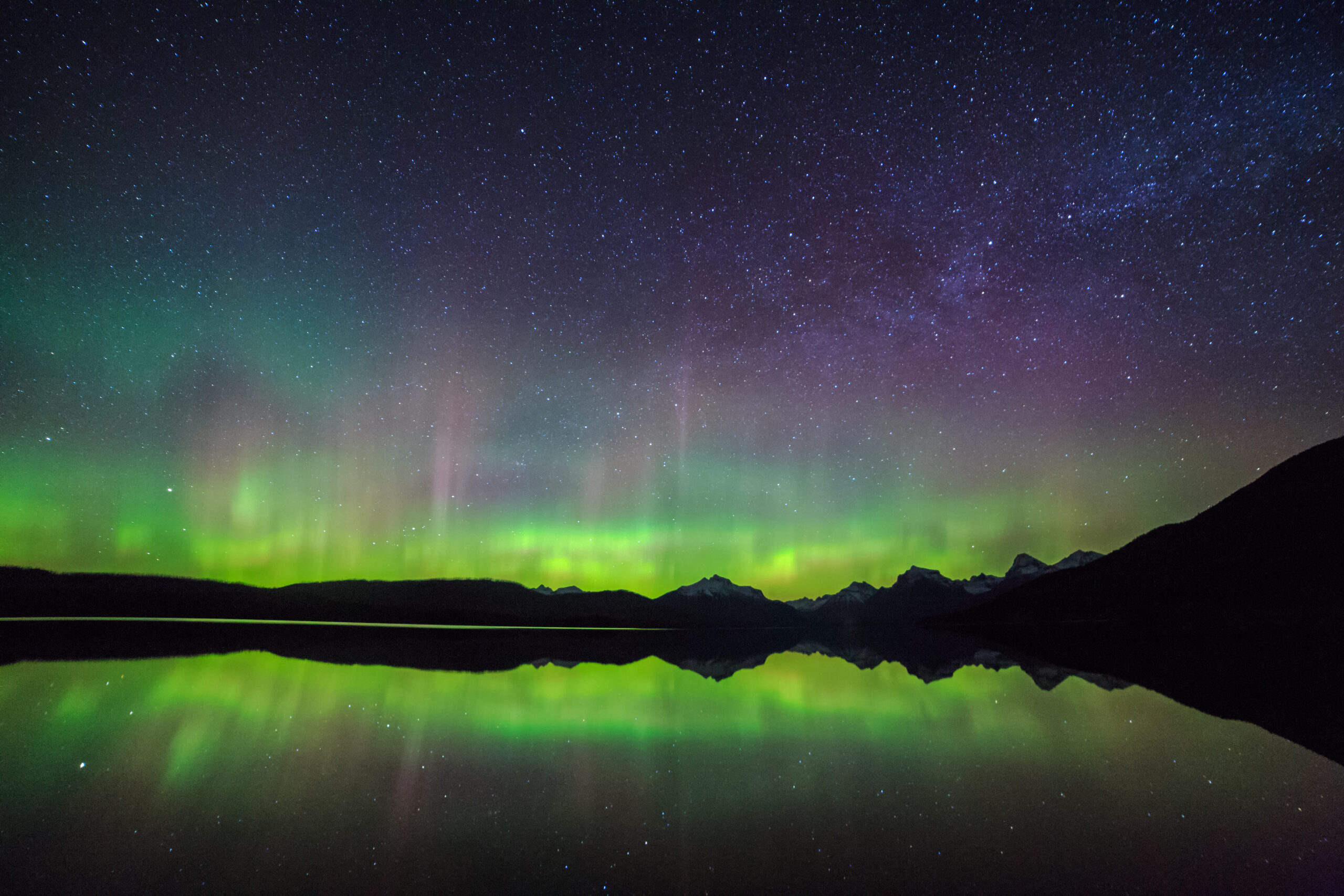This nighttime photograph beautifully captures the Aurora Borealis, or Northern Lights, with vibrant hues of green, yellow, purple, and blue, spanning across the sky above a tranquil lake. The clear, crystal waters mirror the ethereal lights, creating a flawless reflection that doubles the stunning visual effect. In the distance, the silhouette of hilly mountains adds depth to the landscape, also reflected crisply in the glassy surface of the lake. The sky is dotted with countless stars, their light mirrored subtly in the water below. A gentle purple haze crowns the Northern Lights, adding an extra layer of atmospheric beauty to the scene. The entire image is a breathtaking symphony of natural elements, with no text to distract from the serene and awe-inspiring vista.